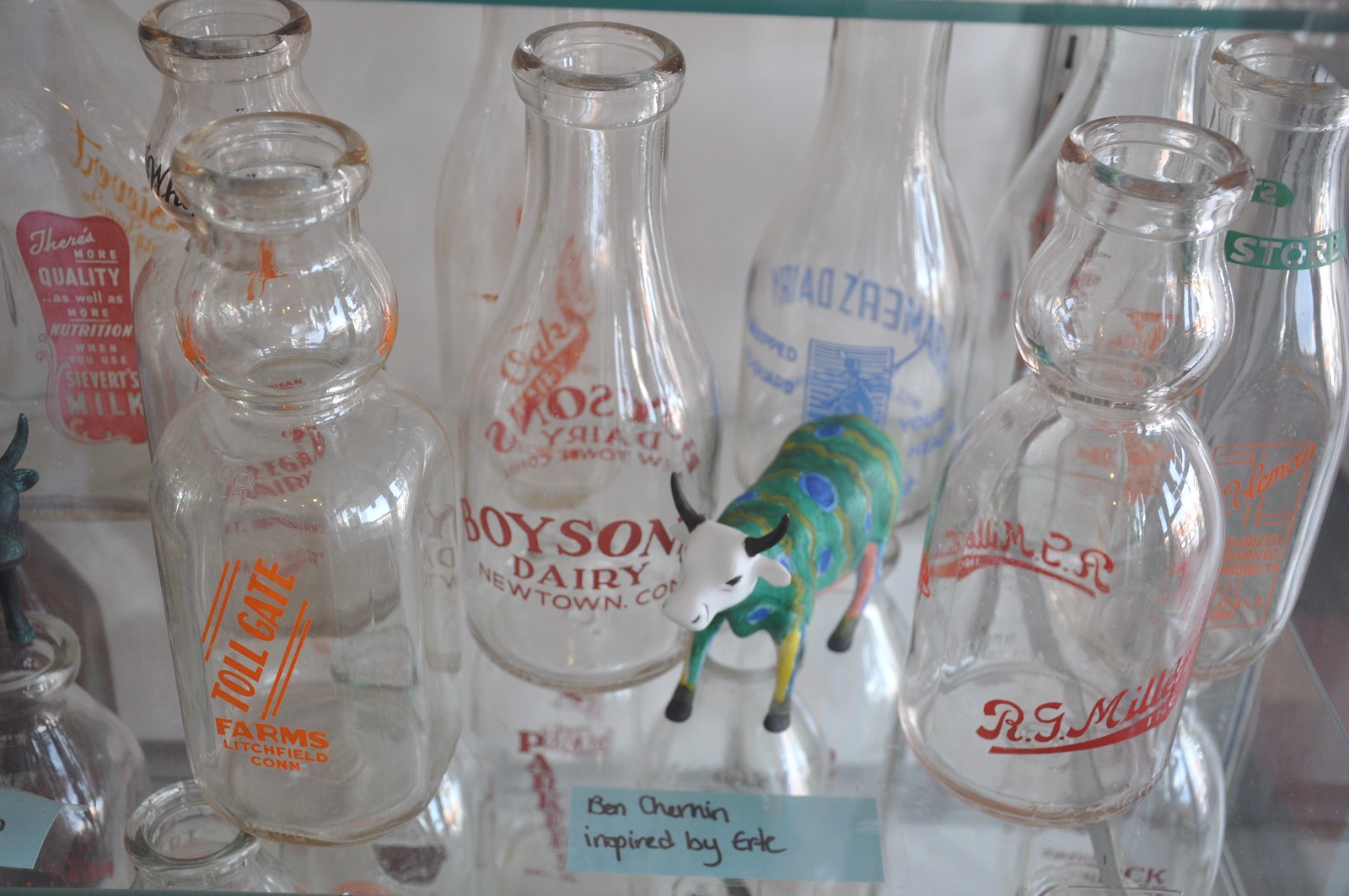The color photograph, in landscape orientation, depicts a collection of about eight vintage glass milk bottles arranged side by side on a glass shelf. The bottles are labeled with names like "Boysen Dairy," "Ardre Miller," and "Tollgate Farms Litchfield Connecticut," suggesting an antique or dairy museum setting. In the center of these translucent containers stands a vividly painted figurine of a cow. The cow’s head is white with black horns, while its body features swirls of green, blue, red, and yellow, including a significant blue spot on its back. A small handwritten note, placed in front of the cow, reads "Ben Chernin, inspired by Erté." The photograph captures the arrangement with a touch of representational realism.